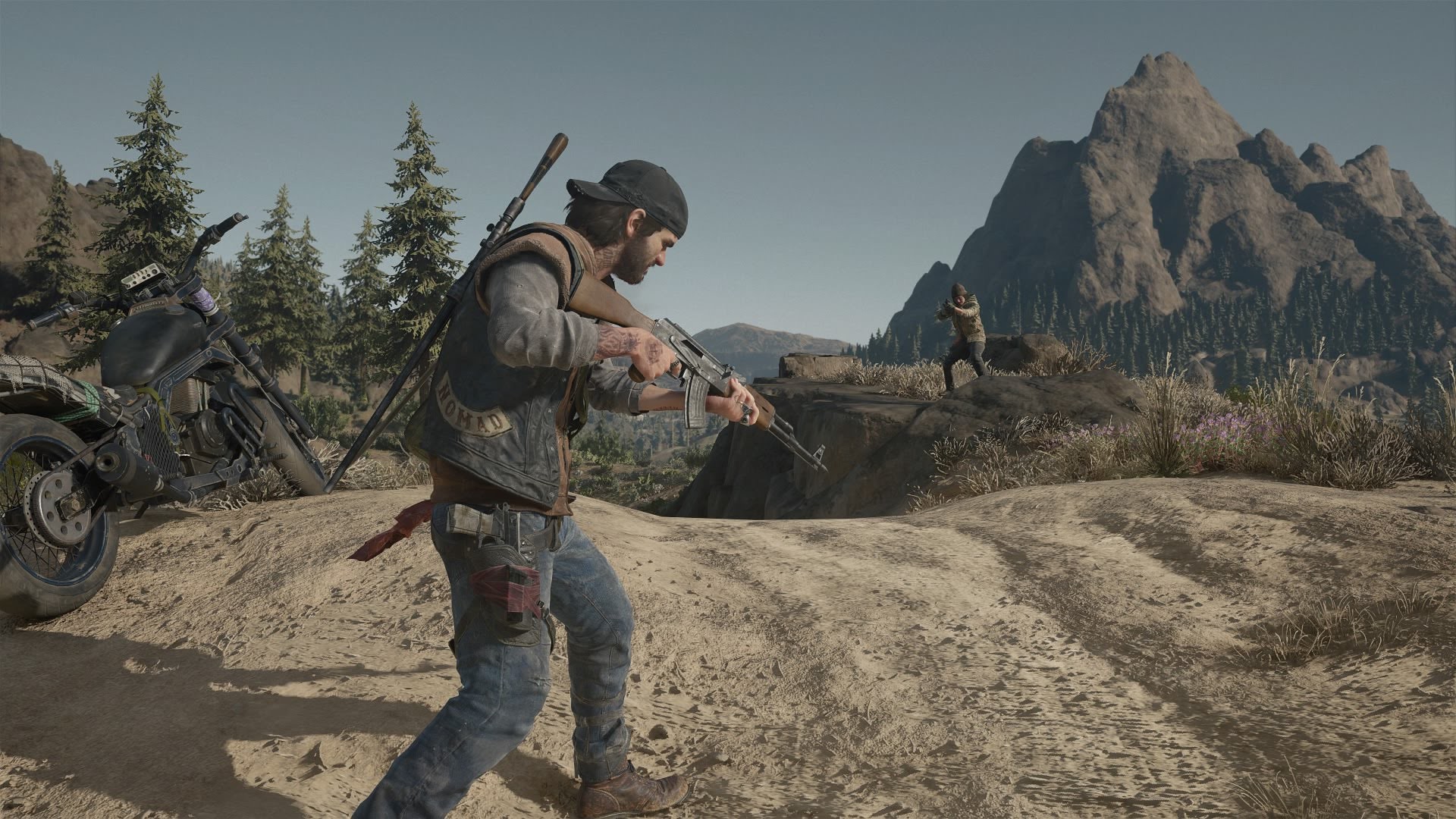In a highly realistic screen capture from a video game, the focus is on two Caucasian men. The man in the foreground is larger and wears a dark baseball cap, sporting longer dark brown hair and a beard. He dons a beige semi-circle patch on his vest that reads "Nomad," blue jeans, and brown hiking boots. Equipped with a thigh holster, and carrying an automatic rifle pointed towards the ground, he bends slightly forward. Additionally, he has another weapon, possibly a knife, strapped on his back.

In the background, another similarly dressed character crouches on a hilly cliff area, aiming at the primary character. Both characters inhabit an arid, scrubby landscape on a cliff, surrounded by larger pine trees on the right. A fat tire, low rider-style black motorcycle sits to the right of the main character, contrasting against the environment. The scene is lit by a clear blue sky, casting shadows that fall to the left of the main character. Tall mountains rise in the distance, adding to the rugged, outdoor setting.